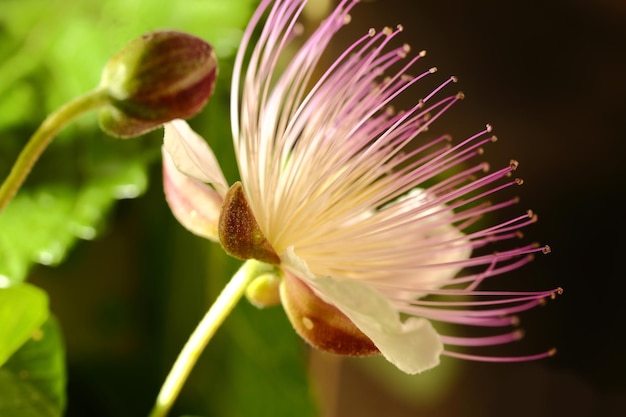This close-up image features a vibrant flower with a light green stem, exhibiting a stunning bloom of purple and white hues. The flower is distinguished by its unique structure where traditional petals are interspersed with long, thin stems that start white at the base and gradually transition to a darker pink, ending in yellow tips. Below the bloom, there's a conspicuous brown part, possibly a leaf. Adjacent to this flower is a bud, yet to open, also supported by a green stem. Both flowers are oriented towards the top right of the frame. The background is predominantly filled with large green leaves on the left side, while the right side fades into a brown backdrop, showcasing a rich array of colors and textures.